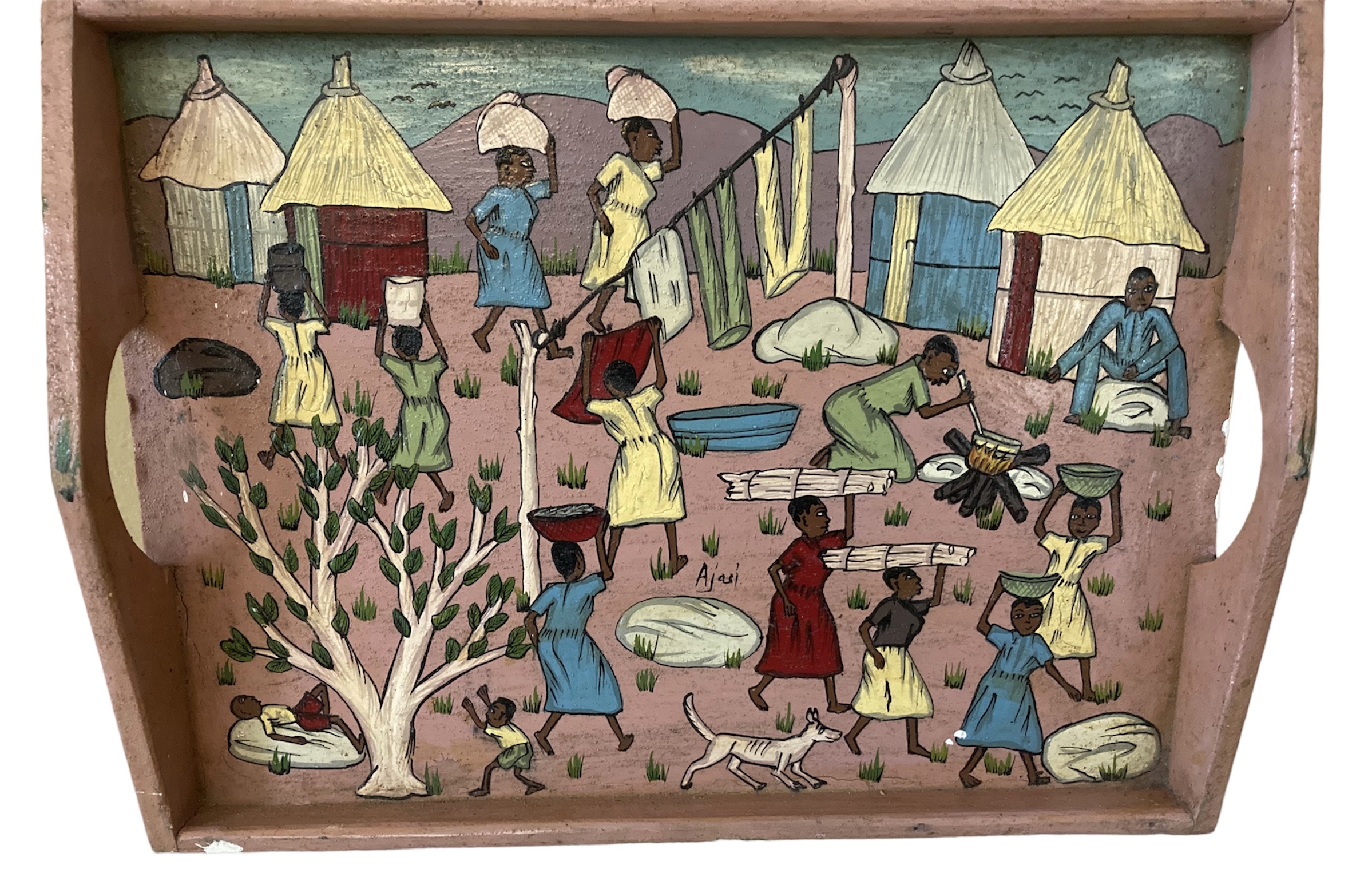The image depicts an old-looking wooden serving tray, possibly repurposed from a cutting board, with sidewalls and raised handles for easy carrying. The entire tray is painted in a tan, light reddish-brown color. It features a detailed and vibrant painting of an African village. The scene includes multiple round huts with straw-covered roofs in hues of gray, yellow, burgundy, and blue, positioned in the upper corners of the tray. 

In the center, two tree posts with a clothesline strung between them display a red blanket, pants, and other garments drying in the sun. Scattered throughout the depiction are villagers, primarily women dressed in colorful attire such as green, blue, and yellow dresses. Many of these women balance items on their heads, including timber, round green bowls, and bundles of sticks while others are involved in various activities—stirring a pot over a fire, carrying water pots, and hanging clothes to dry.

A single man dressed in blue clothes sits on a rock on the right side of the tray, observing the bustling scene. Children play under a verdant white tree in the lower left corner, accompanied by a white dog. The intricate and dynamic artwork transforms the serving tray into a captivating decorative piece, showcasing everyday life in an African village.